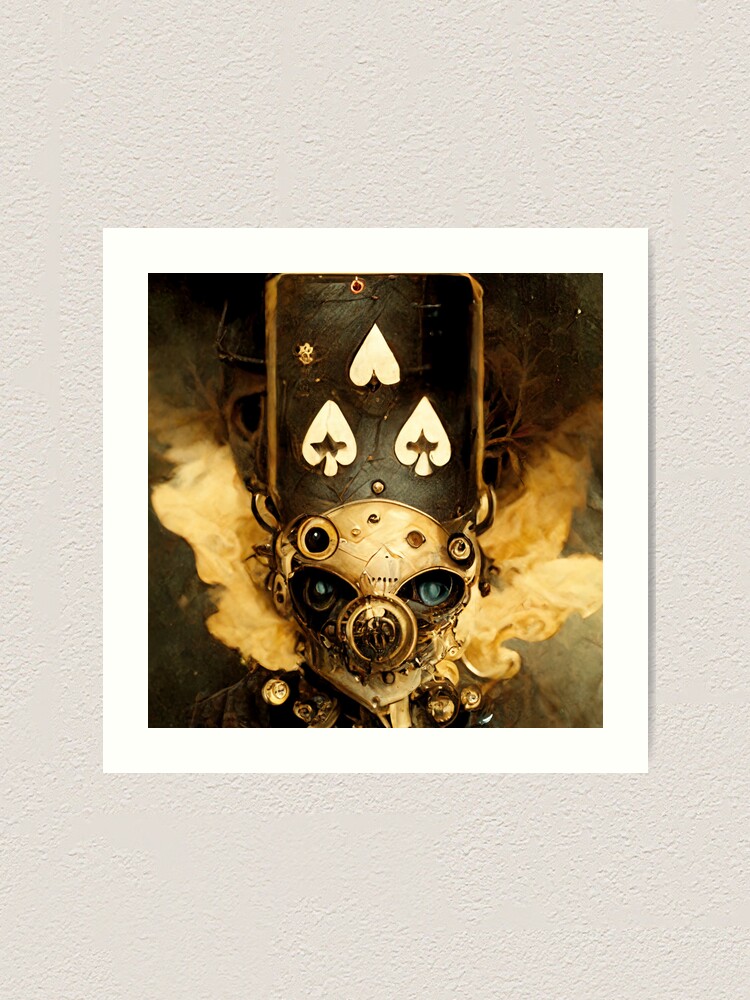The image is an abstract piece of art with a distinctive steampunk aesthetic. It features a metallic, skull-like mask with large, dark eyes and a circular nose. The mask is topped with a black miter, which has three upside-down heart shapes, two of which resemble spades, while the center highest one is stemless, and all are white against the black background. Smoke or possibly flames seem to emanate from behind the mask, enhancing its mechanical, steampunk feel. The color palette mainly consists of metallic browns, golds, and dark grays, with some elements of blue in the eyes and hints of lighter tan. The overall impression is one of a gas mask with robotic dog-like features and a hint of clownish attire, making the image quite abstract and visually compelling. The background of the image is white, and there are no texts.